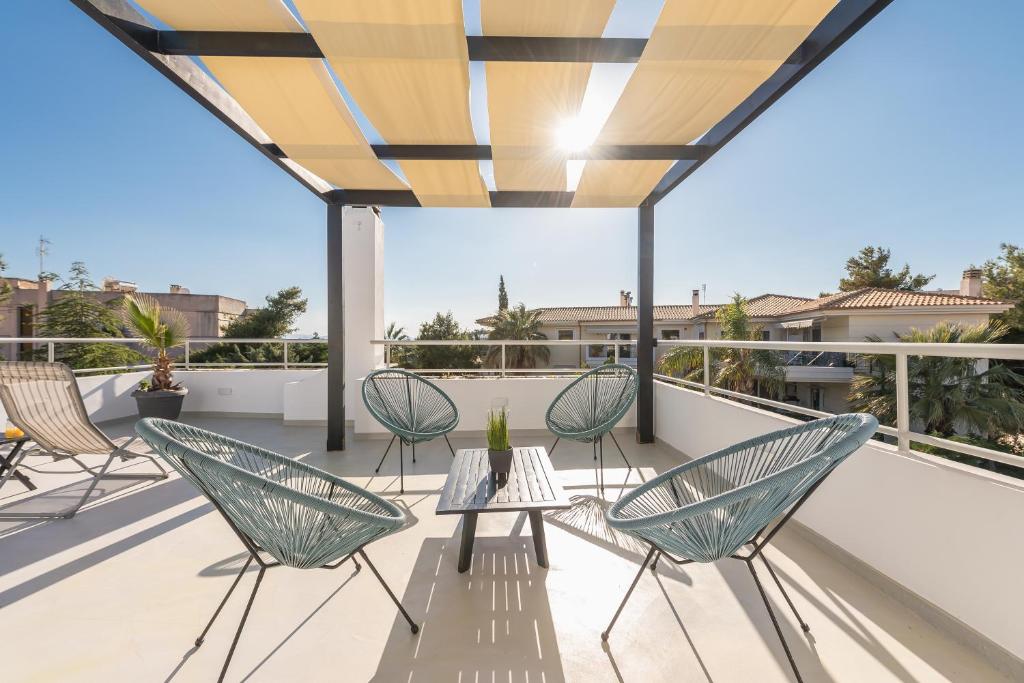This detailed photograph captures a sunlit rooftop patio. The rooftop floor and surrounding low walls are pristine white, extending up about two feet with an additional guardrail featuring two horizontal bars all around. Dominating the left corner of the patio is a large planter housing a tall palm tree. Below this planter, we spot a beige lounge chair, reminiscent of those found poolside, made of thin fabric.

At the patio's center, there are four circular chairs, each standing on four legs, positioned in a square formation. Between these chairs, a rectangular coffee table with wooden slats is centered, casting patterned shadows on the white floor below. Atop the table sits a small planter with a modest plant. Suspended above the seating area is a woven sunshade with gaps that let sunlight filter through, hinting at a light, airy shelter.

In the distance, the view expands to the rooftops of nearby homes and a mix of palm and leafy trees, enhancing the open, elevated ambiance of this space.